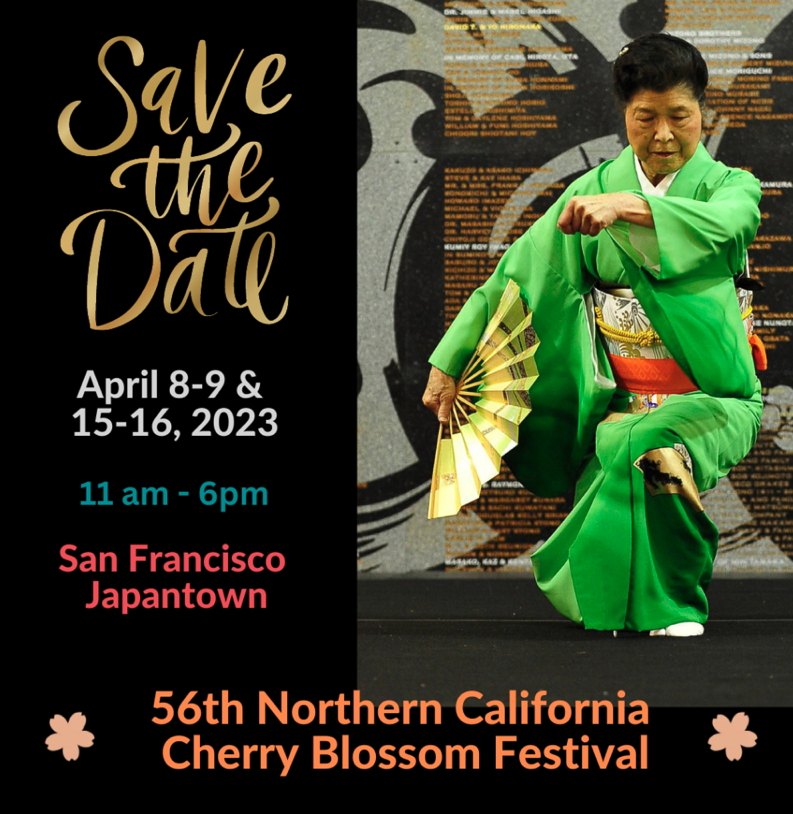This is a detailed poster for the 56th Northern California Cherry Blossom Festival. On the right side of the image, a Japanese woman, possibly in her 60s or 70s, is depicted dancing. She wears a light green kimono with a silver and white pattern, adorned with an orange waistband and yellow ropes. Her black hair is styled in a bun at the top of her head. She holds a yellow paper fan in her right hand. The background features a wall with small, unreadable writing. To her left, the text against a black background reads "Save the Date" in gold. Below, the dates "April 8th-9th and 15th-16th, 2023" are written in white. Further down, it states "11 a.m. to 6 p.m." in blue text and "San Francisco Japantown" in red. At the bottom of the poster, "56th Northern California Cherry Blossom Festival" is written in orange, flanked by illustrations of cherry blossom petals in the corners.